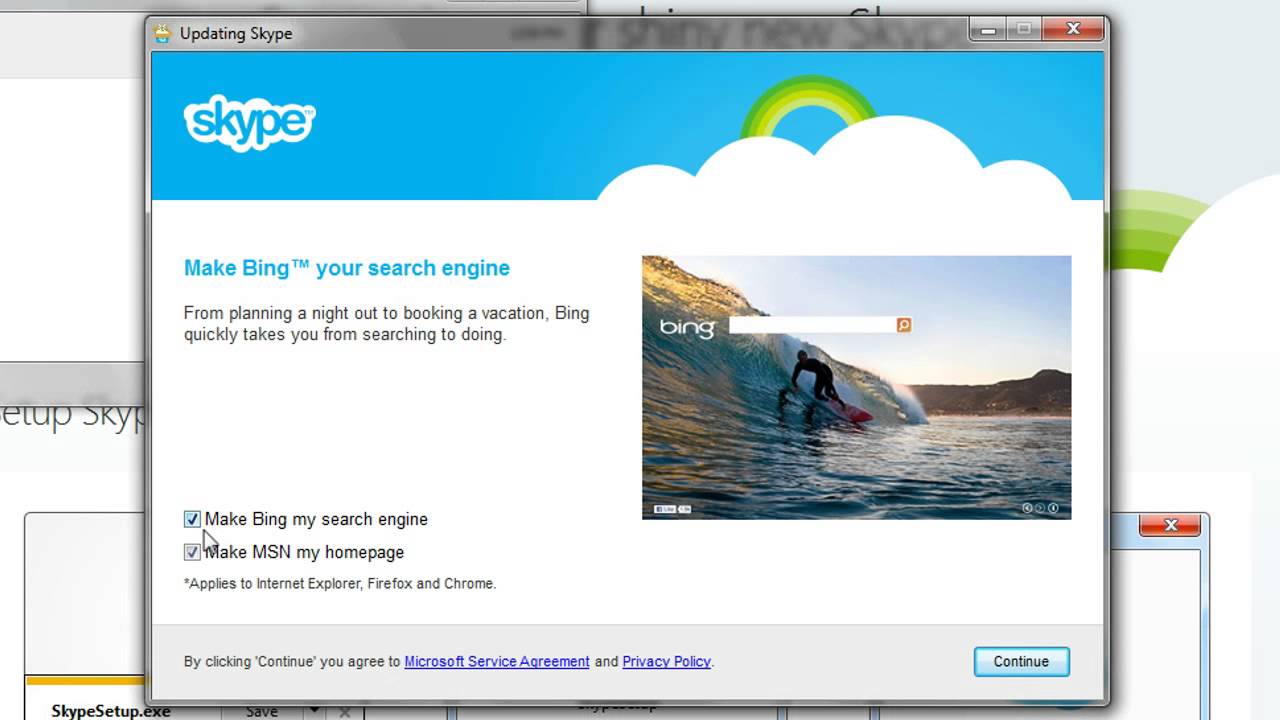In this horizontally-oriented rectangular image, we see a screenshot of a software update prompt for Skype. The prompt features a light gray outlined box with a gray banner at the top left corner, indicating "Updating Skype." To the right of this, though slightly blurred, are the words "Shiny new Skype." Below the banner, there is a prominent thick blue box on the left side, featuring the word "Skype" in blue text within a white cloud design. Beneath this is a white box containing blue text that reads, "Make Bing your search engine." Directly below, in dark gray text, is the sentence: "From planning a night out to booking a vacation, Bing quickly takes you from searching to doing." To the right of these texts appears a colorful rectangular photo of a man riding a wave on a surfboard. In the upper left corner of the image, there is a search bar with the word "Bing" in white text to the left, matching the theme of encouraging Bing search usage.